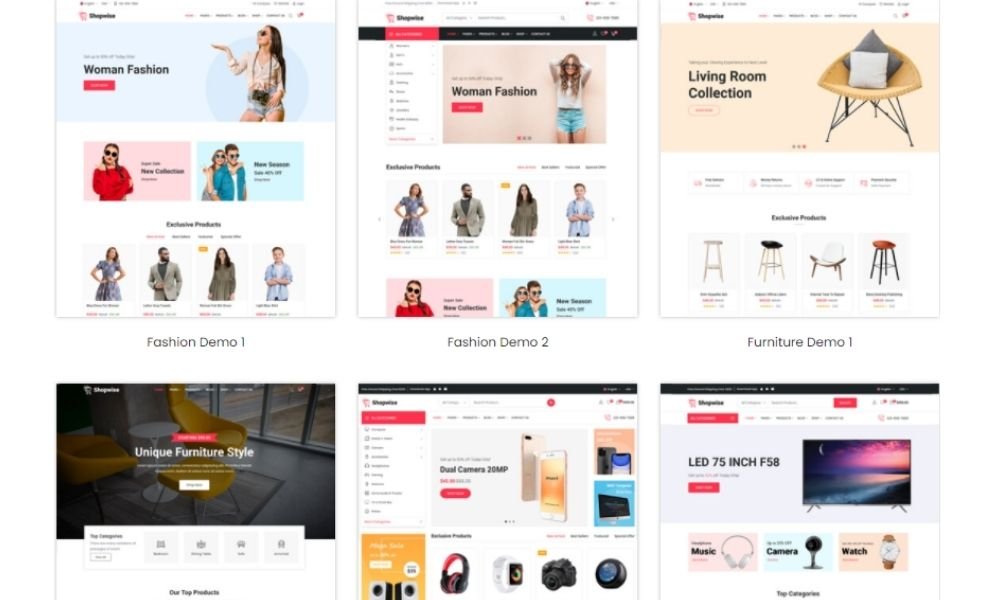In this composite image, we observe six distinct yet similar website layouts, each presented in individual squared boxes. 

1. **Top Left (Fashion Demo One):**
   - The header features a vibrant image of a woman at the center, clad in short blue jean shorts, accessorized with either a purse or a camera around her neck, and wearing sunglasses. 
   - To the left of the woman, the text reads "Woman Fashion."
   - Below, two smaller boxes: one pink with a woman, and one blue showcasing both a man and a woman.
   - At the bottom, four profile boxes display individuals dressed in various outfits. From left to right: a woman in a blue dress, a man in a gray suit, a woman in a green dress, and a man in a blue shirt.

2. **Top Middle (Fashion Demo Two):**
   - This section mirrors the layout of "Fashion Demo One." However, the top image features a different woman who faces the camera, dressed in light blue shorts, with her arms resting on her head.
   - The lower portion remains consistent with the previous layout, retaining the same smaller boxes and profile images.

3. **Top Right (Furniture Demo One):**
   - Diverging from the fashion themes, this box is labeled "Furniture Demo One" and highlights a light brown chair as the central image.

The image sequence continues similarly with other demos not described in detail yet but likely following the pattern of themed boxes showcasing respective designs and layouts. 

The intricate details and structured arrangement suggest that these are likely mockups or previews of website designs, each tailored to distinct themes such as fashion and furniture.